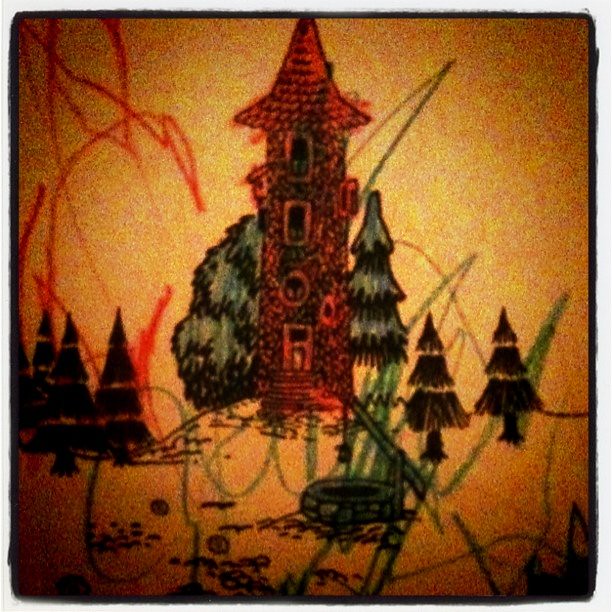The image features a detailed drawing set against an orangish-yellow, speckled background. Dominating the center of the picture is a four-story tower with a red pointed roof. The tower's facade is rendered in alternating red and black colors. Moving from the top down, the tower displays two rectangular windows, a circular window, and finally, a door accessed via a small flight of steps.

Flanking the tower, several trees add to the scene's charm. To the right of the tower, there are three tall pine trees, their shapes distinctly conical. On the left side, a leafy tree stands beside another set of three pine trees, mirroring the arrangement on the right.

The tower stands proudly atop a hill, which is sketched in black. In the foreground, in front of the tower, a green stone well adds another point of interest. The entire scene is animated with various scribbles scattered throughout, featuring splashes of red and green, contributing a touch of whimsical chaos to the structured illustration.